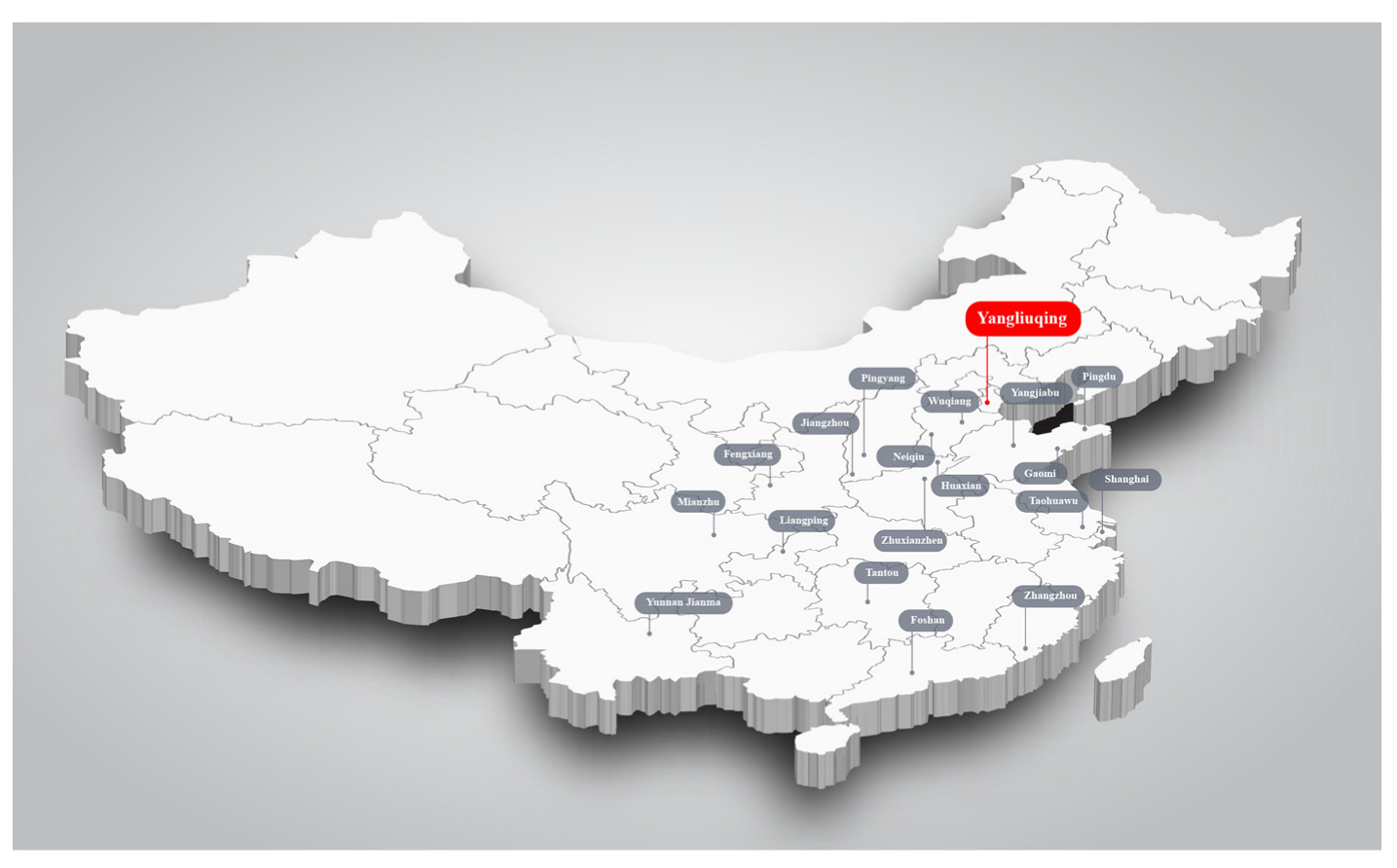The image depicts a three-dimensional map of mainland China, including Taiwan, set against a gray rectangular background. The map itself is white with thin gray lines delineating the provinces, each labeled with white text inside tubular-shaped, rounded-end rectangles. Some of the notable regions labeled include Shanghai and other provinces, though some names are harder to pronounce. Distinctly, there is a red label with the name "Yangxinjing" highlighted more prominently, connected by a red line to its designated location. The map's surface appears raised, giving it a three-dimensional cutout effect, and the overall layout includes irregular borders and concave indents, adding to its detailed topographic depiction. Small islands surrounding China are also visible, emphasizing the geographical context.